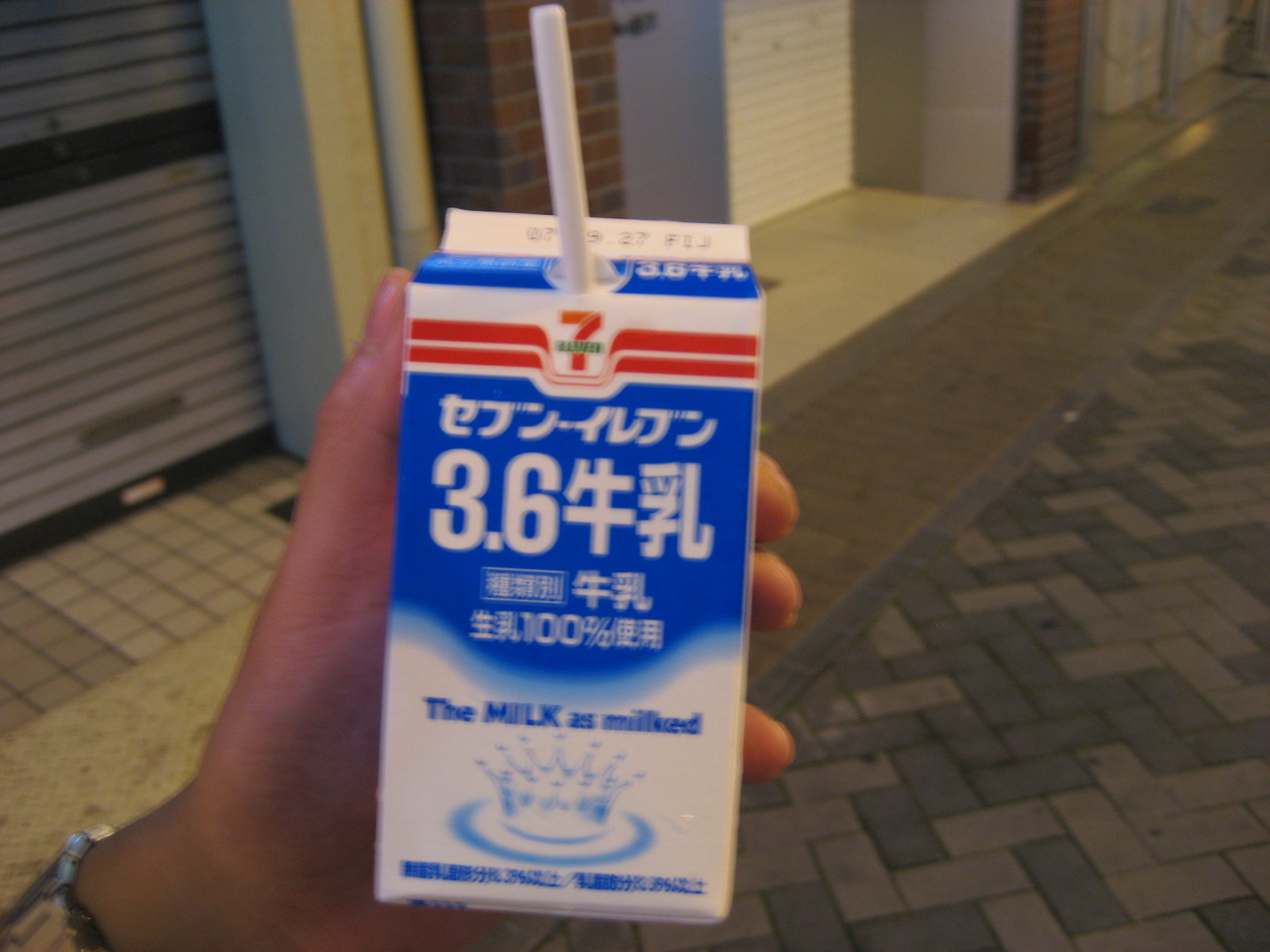The image depicts a close-up of a small white carton of milk held in a light-skinned hand adorned with a silver watch. The photograph shows the person standing on a herringbone-patterned concrete brick sidewalk. The background reveals a brick building with both regular and white-painted bricks, along with several roll-up garage-style doors that may belong to a storage shed. The milk carton, slightly left of center in the image, features a design with a red "7" between two red lines and the green text "11" across the top. Below this, there's a patch of blue containing white writing and Chinese characters, including the number "3.6." Further down, the carton has the words "the milk" followed by additional text and a blue crown with a blue circle underneath. A white straw sticks out from the top of the carton.